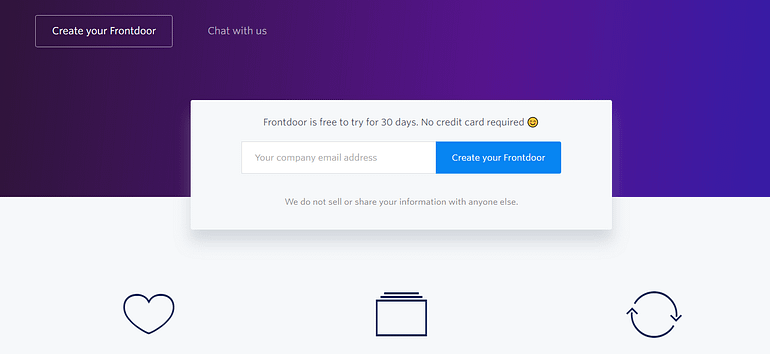The banner on the webpage features a vibrant gradient backdrop transitioning from blue to violet. In the top left corner, two selection buttons are prominently displayed: one within a white rectangle, labeled "Create Your Front Door," and another adjacent button that reads "Chat with Us." 

Centrally situated within the banner, a pop-up message announces a special offer, stating, "Front Door is free to try for 30 days, no credit card required," accompanied by a cheerful yellow smiley face emoji. Below the message, there's a field for users to enter their company email address and create their Front Door account.

At the bottom of the banner, a small gray disclaimer assures users, "We do not sell or share your information with anyone else." Additionally, the bottom left corner features a heart icon, while the center of the bottom edge displays a purple rectangle adorned with two horizontal lines on top. The bottom right corner is marked by two arrows curving around each other, symbolizing refresh or reload.

This detailed layout offers an intuitive user experience, encouraging engagement with clear navigation options and providing reassurance about privacy.